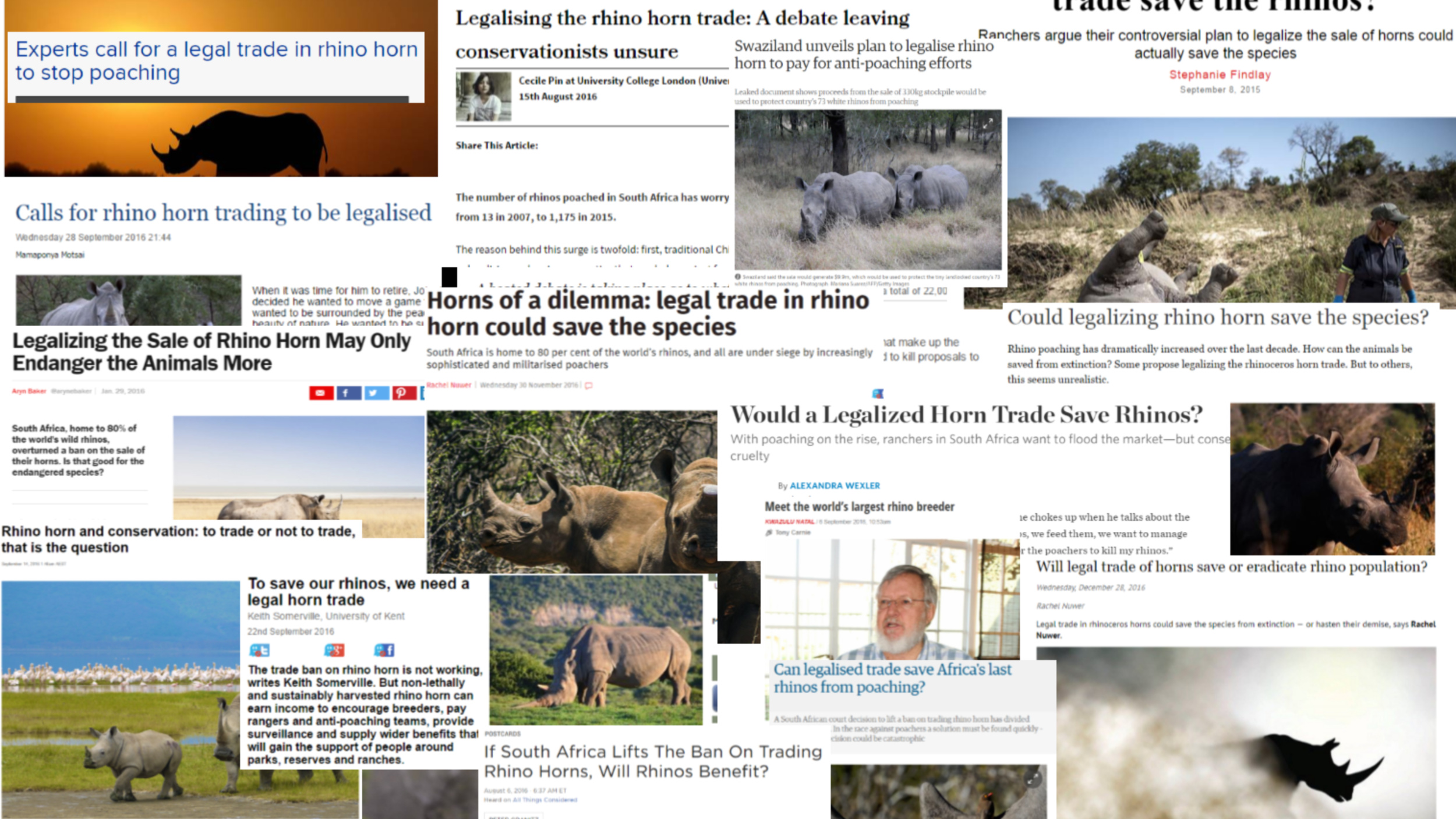A collection of articles provides a deep dive into the controversies surrounding rhino conservation, specifically the debate on the legalization of the rhino horn trade. Experts argue if allowing legal trade could curb illegal poaching or if it would further endanger these majestic creatures. Opinions diverge on whether lifting the ban in South Africa would benefit or harm the rhino population. Accompanying these articles is a poignant series of images: a striking silhouette of a rhino against a vivid orange sunset, rhinos traversing tall grass that reaches their bellies, a woman watching as a rhino runs into the distance, a close-up of a rhino's face, a detailed shot of a rhino horn, and serene scenes of rhinos grazing. These visuals capture the power, elegance, and vulnerability of rhinos in their natural habitat.